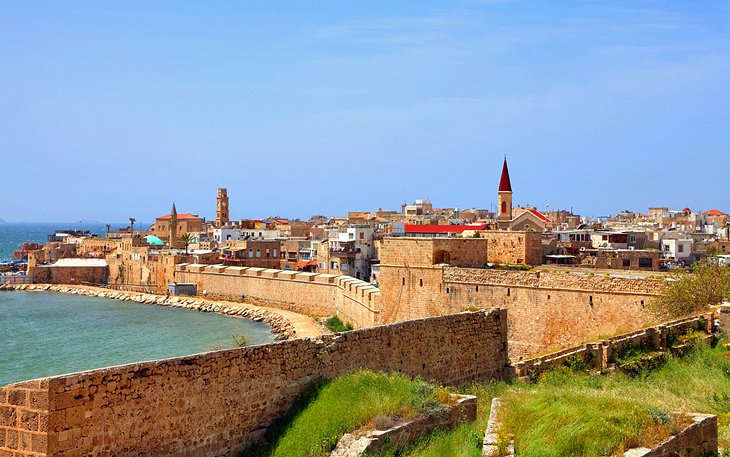This color photograph, taken during daytime with clear blue skies, captures a breathtaking view of an ancient, European coastal city encircled by a massive stone and brick wall. The city is perfectly nestled beside a bay area, with the deep blue of the ocean mirroring the sky above. The imposing walls, in shades of light brownish beige, completely surround the city, with patches of green grass accentuating the earthy tones.

Dominating the cityscape are numerous chapels and cathedrals, their spires piercing the skyline, hinting at the city's rich historical and architectural heritage. The streets within the wall appear bustling with activity, indicative of a busy, vibrant community. The bottom right-hand side of the frame shows a patch of grass, adding a touch of nature to the otherwise heavily built-up area. In the background, the serene water forms a beautiful contrast to the dense, stone-clad urban environment, creating a picturesque scene that blends natural beauty with historical grandeur.